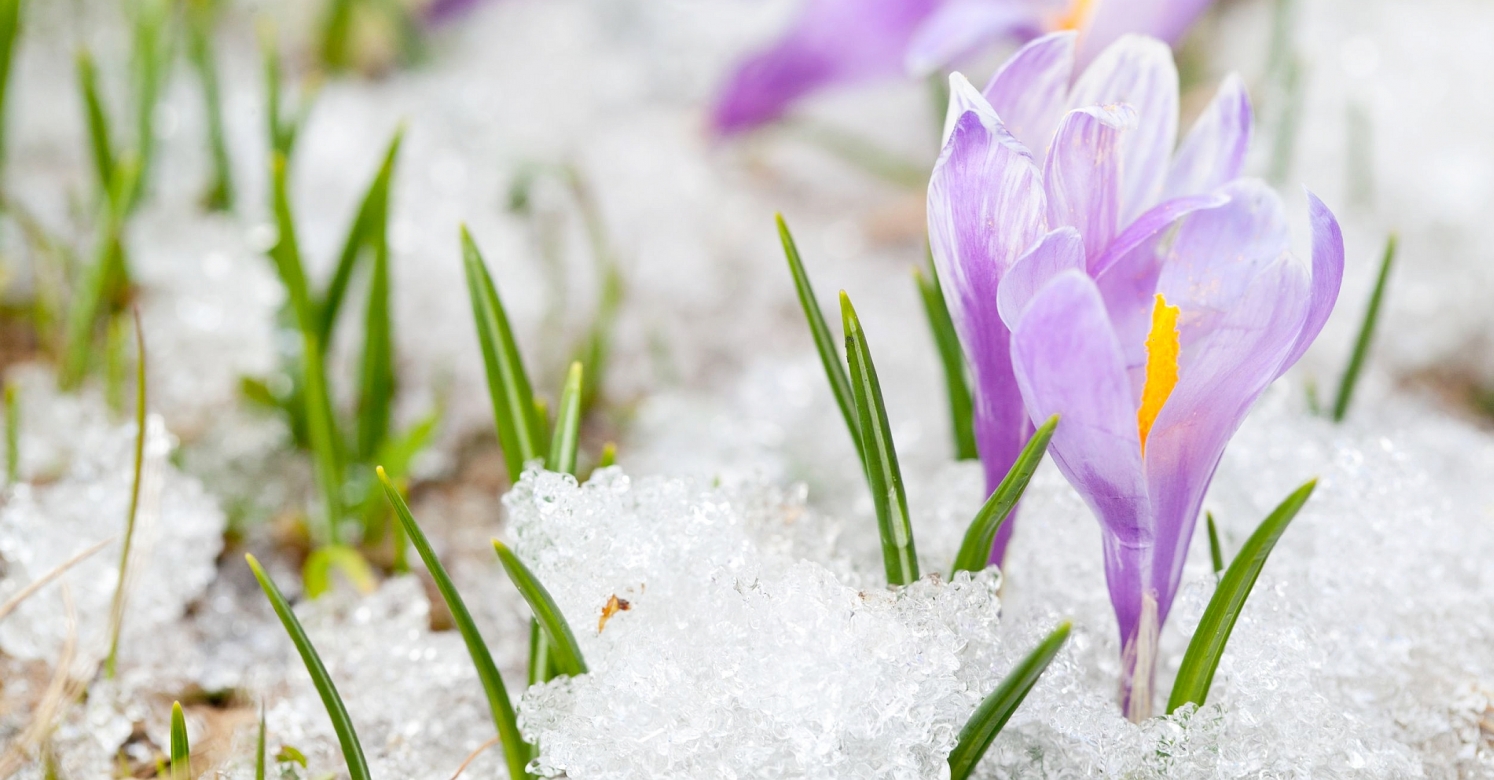This detailed, close-up photograph captures the early springtime emergence of purple crocus flowers bursting through a thin layer of snow and ice. The image is landscape-oriented, with a wider perspective. Dominating the right side are two primary crocus blooms with approximately five light lavender petals each, slightly funnel-shaped, and showcasing bright yellow centers. Thin green leaves accompany these blooms, poking up through the ice crystals. In the background, a third, out-of-focus crocus can be glimpsed, adding depth to the image. The snow on the ground is highly detailed, with clearly defined ice crystals creating a delicate, white backdrop. The focus of the camera is primarily on the lower and right sides, presenting a harmonious blend of light purples, vibrant yellows, tender greens, and pristine whites, epitomizing the very essence of spring as life begins to stir through the thawing frost.